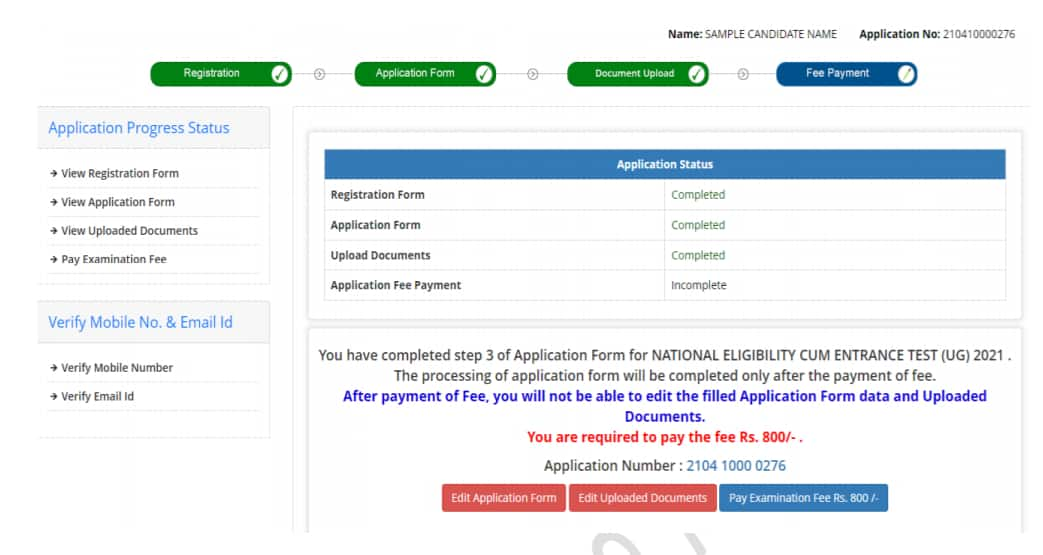The image displays a detailed form with various sections and status indicators. In the upper right corner, there's a label reading "Name: Sample Candidate Name." Adjacent to it, "Application Number: NO: 21410000276" is displayed. Below, a horizontal status bar is segmented into four parts: Registration, Application Form, Document Upload, and Fee Payment.

Beneath the status bar, aligned to the left, are two vertical sections. The first section is titled "Application Progress Status," and the second section is labeled "Verify Mobile Number and Email ID." To the right of these sections, an "Application Status" area is displayed, indicating that all steps—except for the "Application Fee Payment"—are marked as complete. The "Application Fee Payment" remains incomplete.